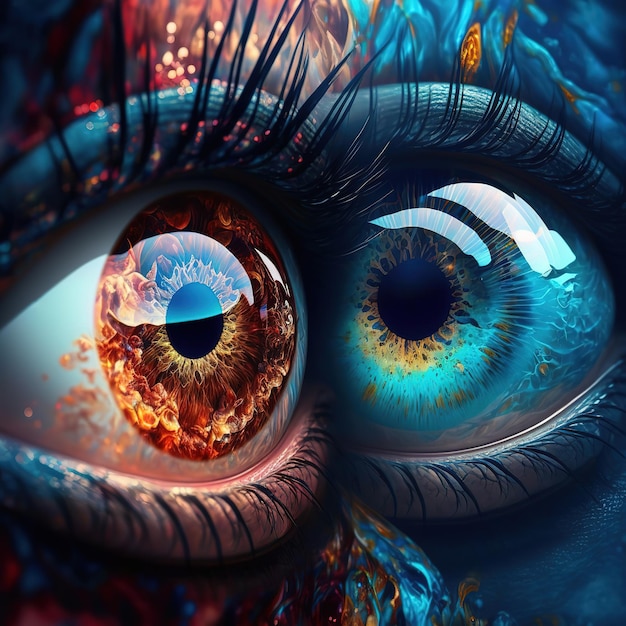This highly stylized, 3D-generated sci-fi artwork features two vividly detailed eyes positioned centrally and almost touching, creating a mesmerizing focal point. The eye on the left is a fiery red, with flames swirling around the white sclera and inside the burning red iris, giving it a smoldering, incandescent quality. Tiny sparks and cinders accentuate the skin surrounding this eye, adding to its intense, ablaze appearance. The eye on the right contrasts with a deep, watery blue hue, resembling the rippling depths of the ocean. The blue iris exhibits subtle hints of orange and brown, adding texture and depth, while the pupil appears abyssal, as if it extends infinitely. The skin surrounding this eye carries an underwater-like essence, complementing its marine theme. Both eyes possess reflective pupils, enhancing their lifelike quality, and are framed by stark black eyelashes. The blending colors—orange and blue—further merge the two eyes into a captivating and uncanny representation of fire and water juxtaposed.